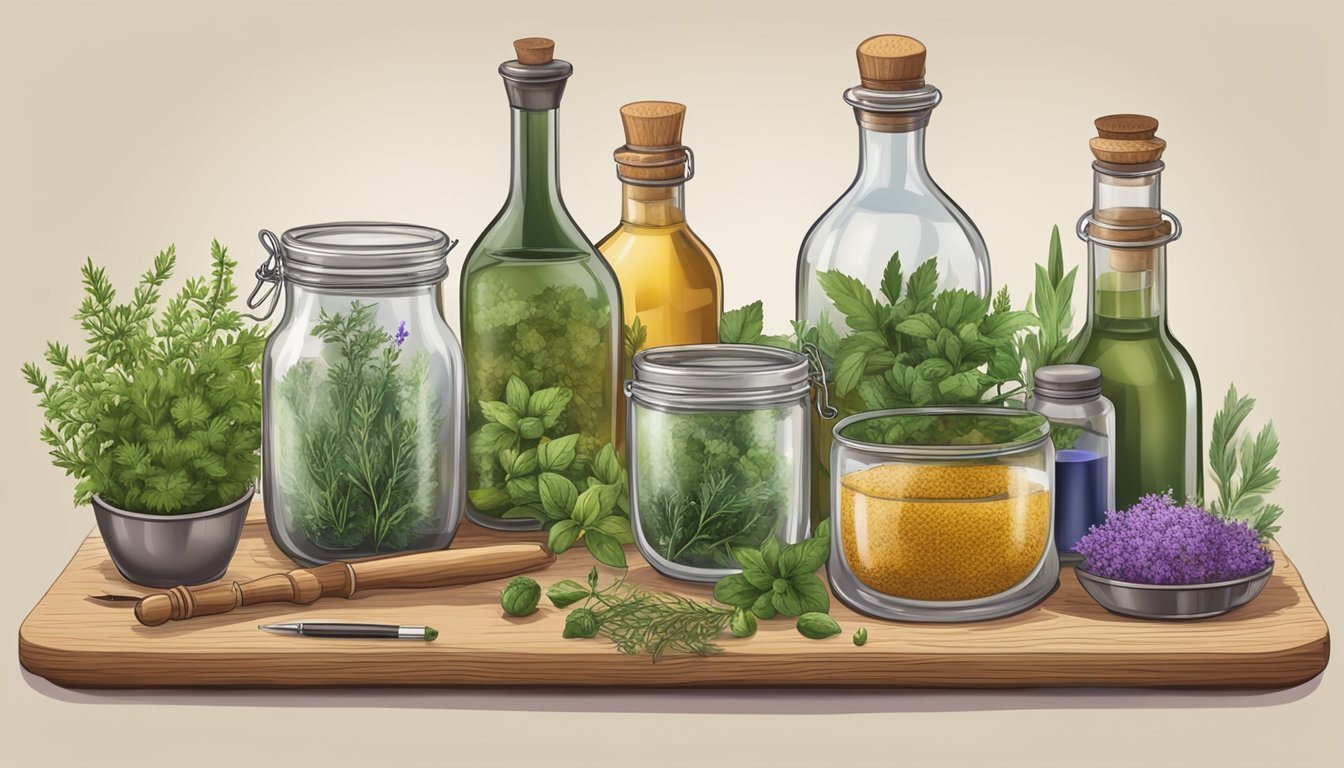The image is a detailed and colorful illustrated painting depicting a wooden board adorned with a diverse assortment of herbs, jars, and bottles. In the foreground, a variety of fresh herbs rest on the wooden surface, alongside a wooden stick and a silver and black handled tool. Further back, there is a mixture of glass jars—some with screw-on lids and others with snap closures—each containing different herbs and liquids in hues of yellows, greens, and blues. A mason jar filled with mustard seeds and another with a screw-top lid are prominently visible. A small bowl of lavender flowers adds a splash of purple. Surrounding these jars, numerous bottles of various heights and shapes are seen, each sealed with cork lids and filled with herb-infused oils, ranging from green to yellow. Completing the scene is a green plant and a silver bowl situated on the wooden board, against a white background.